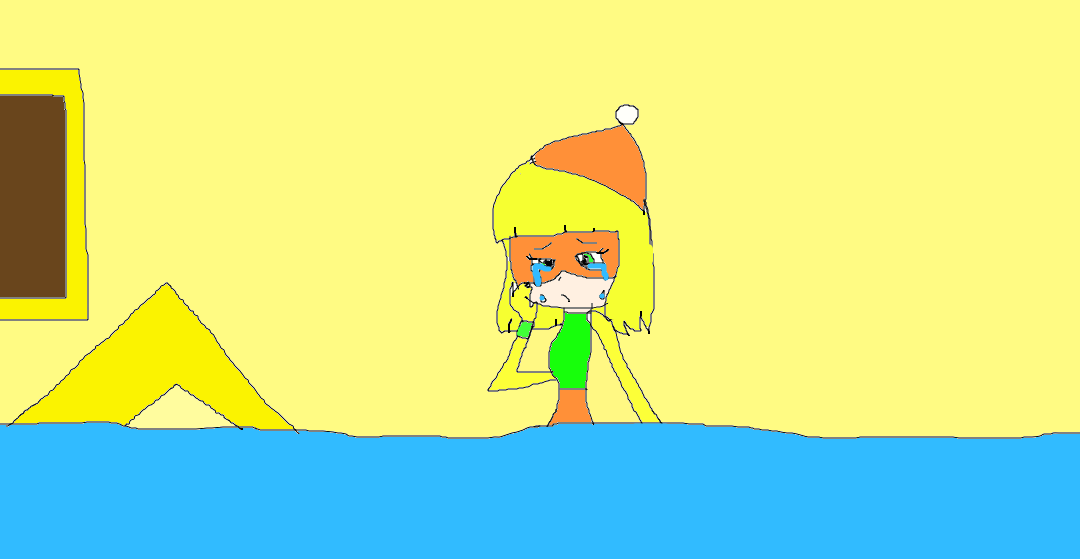This hand-drawn cartoon illustration depicts a young, pixie-like girl with shoulder-length blonde hair and bangs, wearing an orange beanie with a white pom-pom on top, a green blouse, and an orange skirt or dress. She sits waist-deep in a pool of her own tears, emphasizing her profound sadness. Her eyes, accentuated with a mask-like area the same orange color as her cap and dress, weep an almost continuous stream of blue tears. The backdrop is a yellow wall, with a framed picture or window partially visible on the left side. Her skin is tinted orange, and her expressive face, marked by green eyes and a white mouth, underscores the emotional weight of the scene. The flood of tears filling the room vividly portrays her sorrow, creating a striking visual contrast against the yellow and blue color scheme.